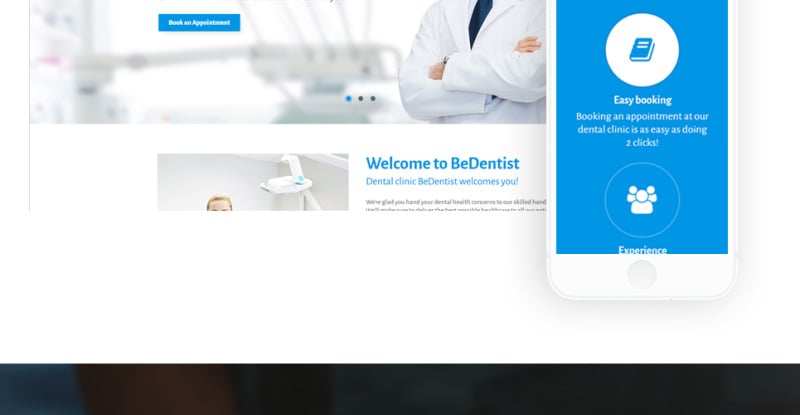The image is a screenshot of a website, prominently featuring a photograph of a doctor. The doctor, a white person dressed in a white lab coat and either a black or blue tie, is standing in what appears to be a medical or dental office, or possibly a lab, with their arms folded across their chest. To the left of the doctor, there is a blue box with the text "Book an Appointment." Below the image, there is a row of three dots indicating page navigation; the first dot is highlighted in blue, and the next two are dark blue, suggesting this is the first of three pages.

Below the navigation dots, bold blue letters read "Welcome to Be Dentist," followed by another message in blue, "Dental clinic Be Dentist welcomes you!" with an exclamation point. Further down, there is an image of another dental office, showing the top of someone's head from the eyes up. Next to this picture, black text is visible but too blurry to read. To the right, clear text reads, "Easy Booking. Booking an appointment at our dentist's clinic is as easy as doing two clicks."